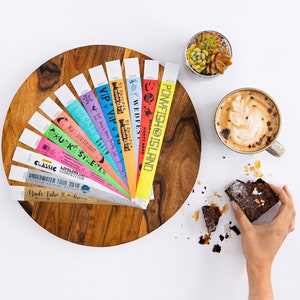This image presents a bird's-eye view of a light gray table or counter displaying a medium-toned wooden tray adorned with a multitude of colorful, narrow rectangular paper strips. The strips, featuring dark wood knots and visible grains, fan out in a triangular arrangement and display various hues, including yellow, red, light blue, orange, turquoise, lavender, light teal, peach, lime green, pink, white, gray, and gold, with printed text like "Pony Fish Island" and "Medieval." To the right, the table hosts a couple of dishes, including a small circular glass dish and a coffee mug filled with hot chocolate topped with whipped cream. A hand entering from the lower right corner holds a partially eaten brownie, completing the eclectic scene of vibrant wristband-like strips amidst inviting refreshments.